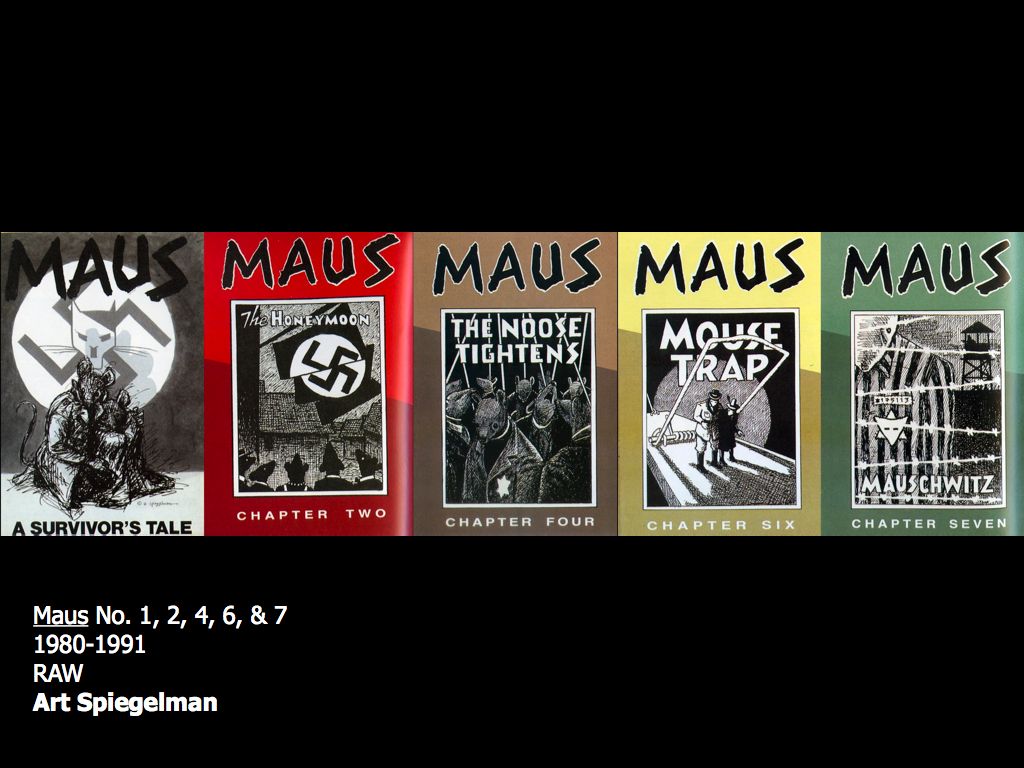The image is a collage of book covers from Art Spiegelman's series "Maus" arranged horizontally against a black background. Each cover prominently features the title "Maus" at the top, with different subtitles and imagery:

1. The first cover, in black and white, titled "Maus: A Survivor's Tale," displays a swastika with a cat's head and people leaning over. 
2. The second cover, with a red background, titled "Maus: Chapter 2, The Honeymoon," also features a swastika and background figures.
3. The third cover, also black and white, titled "Maus: Chapter 4, The Noose Titans," shows pig-faced figures in men's outfits with Jewish stars on their coats.
4. The fourth cover, against a golden yellow background, titled "Maus: Chapter 6, The Maus Trap," depicts two individuals walking in a mousetrap.
5. The fifth cover, with a green background, titled "Maus: Chapter 7, Mauschwitz," shows a person in a striped outfit with a Jewish star, evoking imagery of Auschwitz.

At the bottom left corner, text reads: “Maus #1, 2, 4, 6, and 7 1980-1991 RAW Art Spiegelman,” indicating the publication years and the author's name.